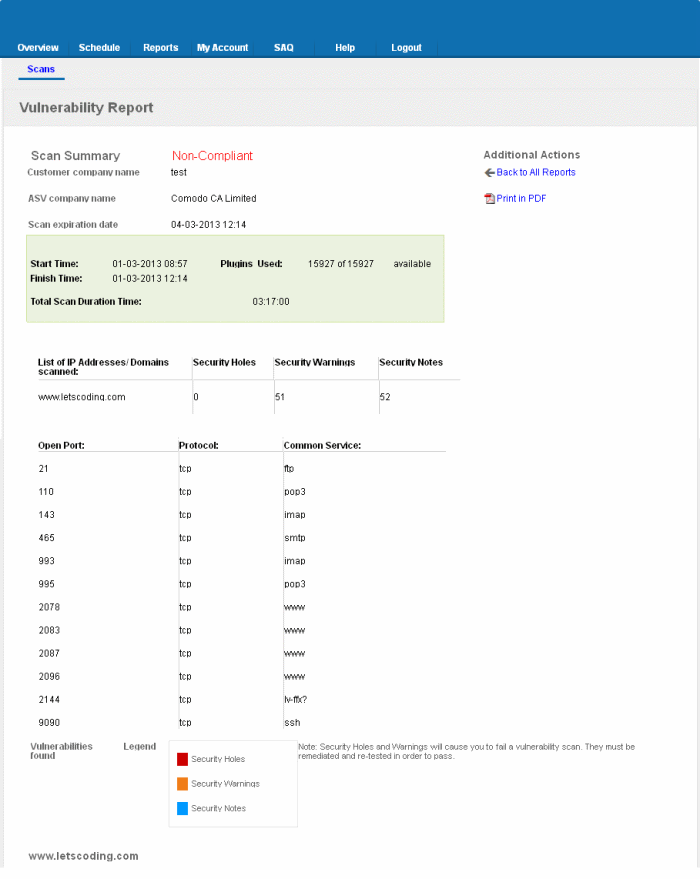This image depicts a detailed vulnerability report page with a primarily white background. At the top, a blue horizontal rectangle runs across the width of the page, containing white text with the navigation options: Overview, Schedule, Reports, My Account, SAQ, Help, and Logout. Beneath this, a gray horizontal rectangle also spans the width of the page. In the top left corner, it reads “Scans” with a blue underline. Below, in bold black text, it says “Vulnerability Report.”

The section opens with a black text heading “Scan Summary” followed by "Customer Company Name," "ASV Company Name," and "Scan Explicit Action Date." The scan summary indicates non-compliance, and a test is mentioned for the customer company name. To the right, there are options for "Additional Actions" including "Back to All Reports" and "Print in PDF."

Further down, a light green rectangle presents key details of the scan: starting time of 01-03-2013 at 08:57, plug-ins used (15927 out of 15927 available), finishing time of 01-03-2013 at 12:14, and a total scan duration of three hours and 17 minutes. 

A list follows, showing scanned IP addresses and domains, such as www.letscoding.com. The security findings include zero security holes, 51 security warnings, and 52 security notes. Specific details like an open port (Port 21) and its associated protocol (Common Service) are also mentioned. 

The report further includes a "Vulnerabilities Found" segment followed by a legend and a note emphasizing that security holes and warnings will cause failure in the vulnerability scan. It points out that these issues must be remediated and retested to achieve a pass status.